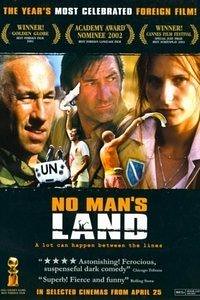The image appears to be a scanned copy or photograph of a DVD cover or a film poster for the movie "No Man's Land." The top section features a black band with text in orange and white, proclaiming it as "The year's most celebrated foreign film." This is followed by award accolades, including "Winner, Golden Globe," "Academy Award Nominee, 2002," and another indistinguishable winner label, each possibly bracketed by golden laurel branches.

Centered in the image is a rectangular photograph of three characters: a man with longish black hair and black stubble stands prominently in the middle; to his right is a woman with dark hair; and to his left is an older man with short, balding gray hair. Directly below this image, set against a black background, is the movie title "No Man's Land," accompanied by the tagline "A lot can happen between the lines."

Further text below includes glowing reviews, such as "Four star astonishing, ferocious, suspenseful, dark comedy" and "Superbly fierce and funny," indicating high praise from critics. Additionally, it notes the movie's selected cinema release date of April 25th. The overall color palette includes black, orange, white, blue, tan, gray, silver, and gold, contributing to the professional and celebratory theme of the poster.